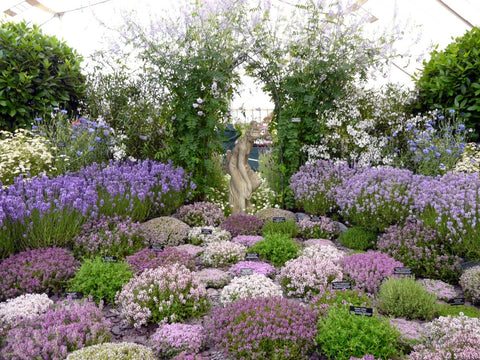The image captures a vibrant, colorful flower garden, possibly situated in a large greenhouse or atrium, under the bright light of mid to late morning. Central to the composition is a statue of a woman, encircled by an arch of climbing greenery. The garden showcases a curated collection of flowers in various shades of purple, from light to dark, interspersed with white and ivory blooms. In the foreground, small, dome-shaped plants with purple and pink flowers are neatly arranged, each accompanied by small information plaques. Taller plants and shrubs with similar flowers frame the flower bed, giving way to larger trees and leafy greenery in the background. Structural supports and glass panels of the greenhouse can be seen above, letting in a stream of sunlight that enhances the vivid colors of the flowers.